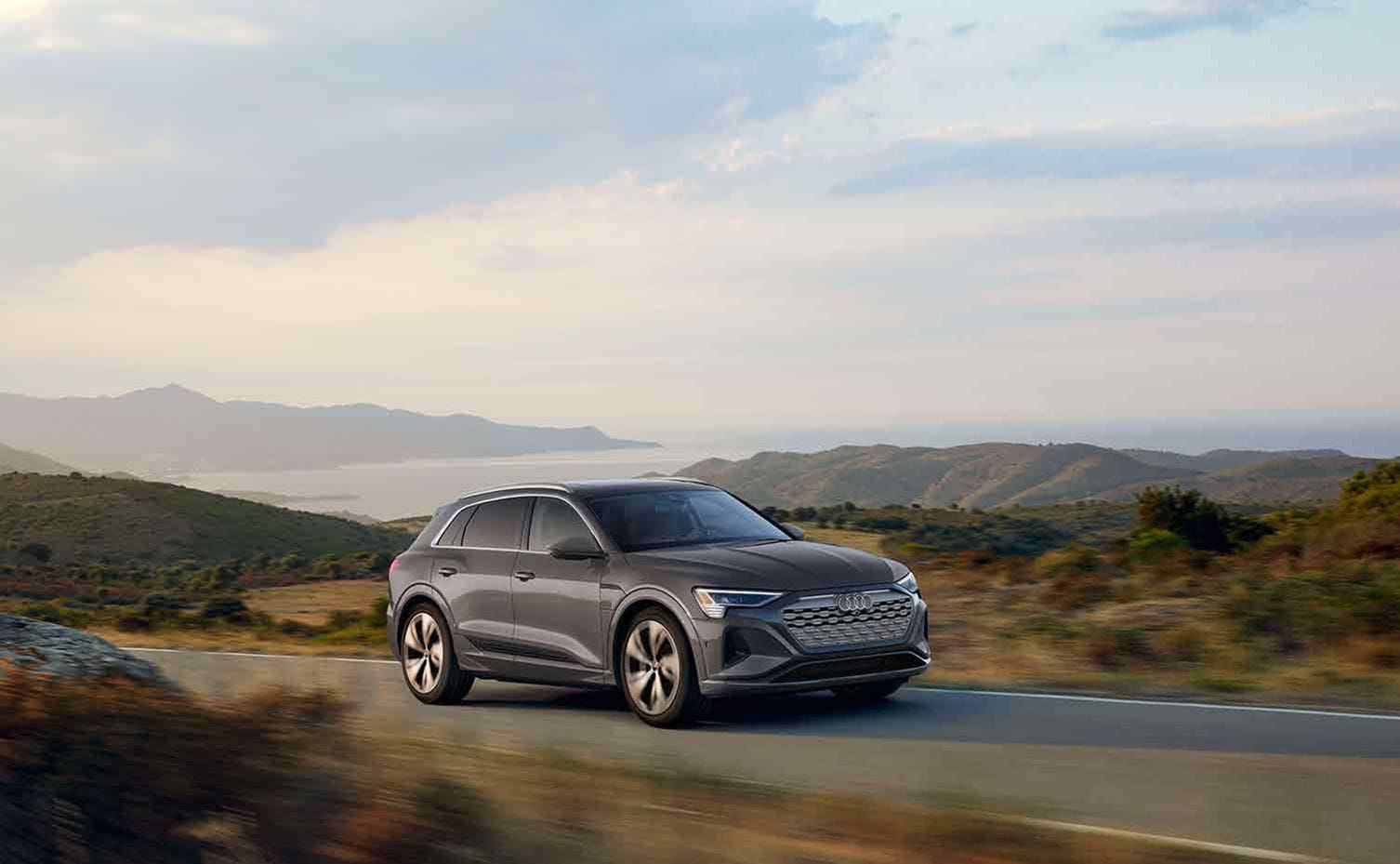The photograph features a sleek silver Audi, either a compact sedan or SUV, driving on a sunlit, gray country road that stretches from left to right near the bottom of the image. The car, recognized by its distinctive Audi symbol on the front grille and stylish headlights, is heading to the right and appears in motion, lending some blur to the small bushes on either side of the road. The scenic background showcases a panoramic coastal landscape with a clear blue sky dotted with white and gray clouds. Nestled between mountain ranges on both sides, the serene ocean glimmers in the distance, enhancing the picturesque setting. The surrounding fields are a mix of verdant greenery and brown patches with scattered shrubs and rocks, creating a harmonious blend of nature's hues. This photo, likely intended for a car advertisement or magazine, captures the essence of a serene yet dynamic driving experience, potentially somewhere reminiscent of California.